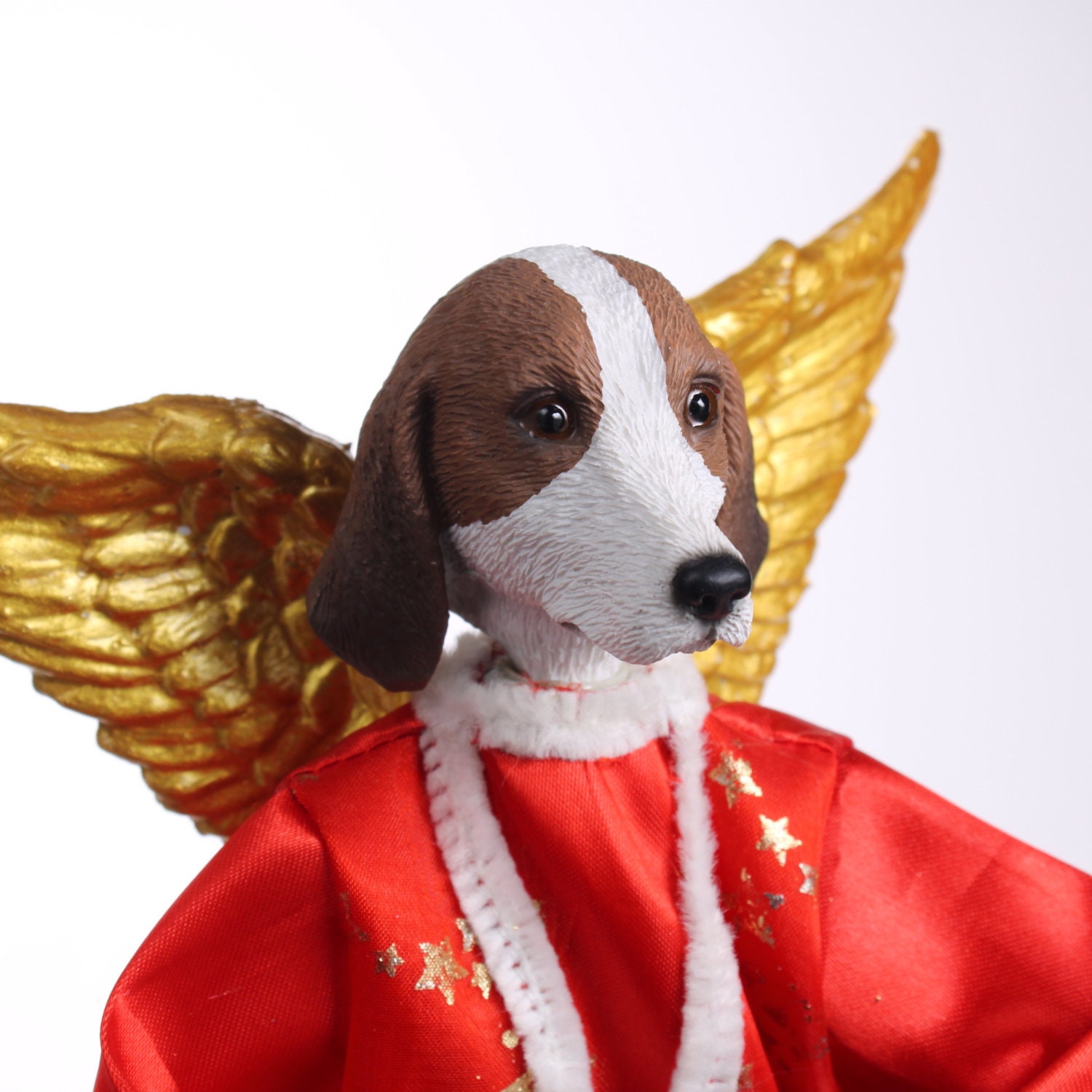The image features the upper half of a small figurine, resembling a beagle, crafted from a material that looks like ceramic. The beagle's head is detailed with a black nose, a white muzzle, and a distinctive white stripe running from the snout over the head. The dog's fur around the sides of its head and around its eyes is brown, and it has long, fluffy brown ears, darker towards the ends. The dog's eyes are dark and glassy, giving an alert expression. It wears a red shirt adorned with gold stars and a thin, white scarf that drapes down the front. Golden angel wings, with feathers lighter than the dog's shoulders, extend from its back, facing up to the upper right and then over to the left. The background is solid white, emphasizing the detailed and colorful features of the figurine.